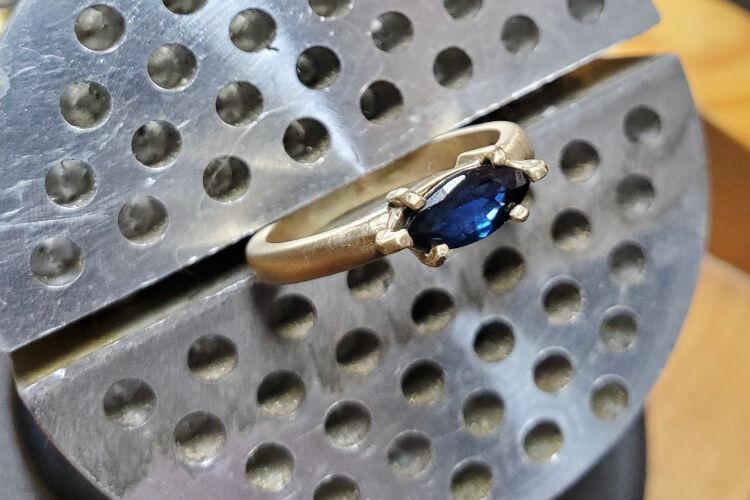This detailed close-up photograph captures a stunning sapphire ring firmly held in a circular silver metal vise. The ring, likely made of gold or brass, features a vibrant, dark blue, oval-faceted sapphire at its center. The sapphire is held securely by six small prongs, with three prongs on either of the long ends of the oval. Light reflecting off the facets of the sapphire adds a vibrant shimmer to the central gemstone, which is the primary focus of the image.

The ring itself sports a simplistic design, with a smooth metal band free of additional detailing. The surrounding vise, which clasps the ring in place, is notable for its circular structure around the edges, small dusty indentations on its surface, and its function of holding the band securely for inspection. 

In the out-of-focus background, a brown wooden surface is subtly visible, enhancing the antique, well-worn aesthetic of the photograph. The chipped and brushed appearance of the vise's metal further conveys a sense of history and usage, contributing to the overall narrative of the ring's craftsmanship and careful scrutiny.